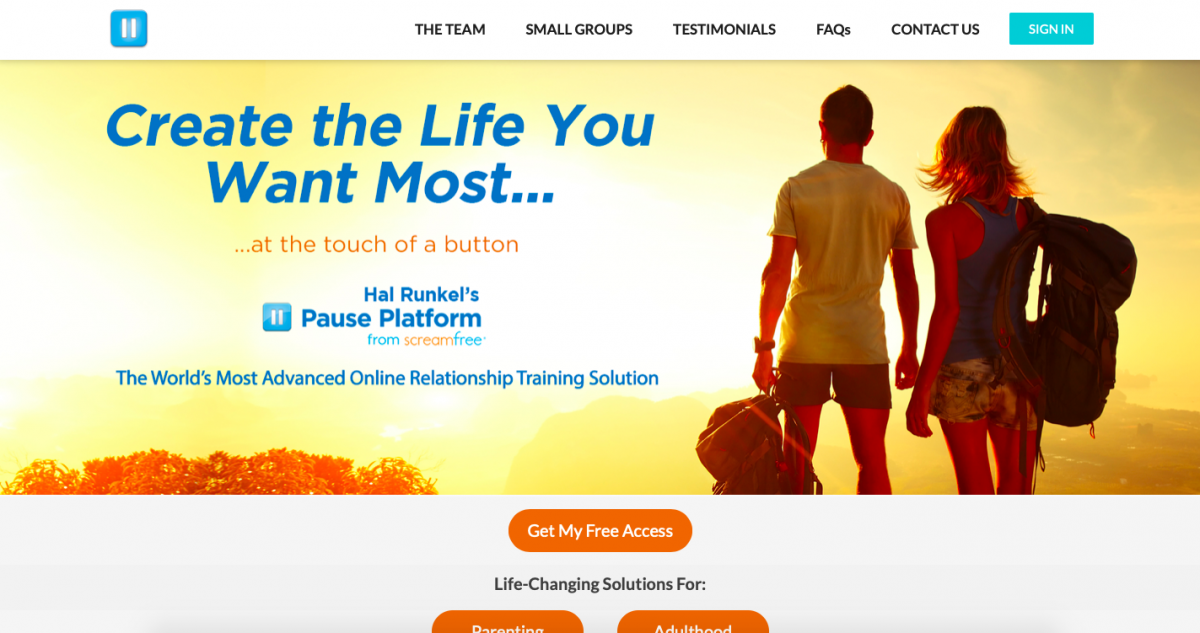This image captures the homepage of a website, prominently featuring a structured layout and vibrant design elements. 

At the top of the image, there's a blue header box with a white pause button icon. Immediately below, there's a navigation bar with menu items in black font, including options such as "The Team," "Small Groups," "Testimonials," "FAQs," and "Contact Us." To the right of these menu items, a teal box with white text invites users to "Sign In."

Below the navigation, a large hero image showcases a man and a woman standing side by side, both wearing casual attire with shorts. The woman, dressed in a blue tank top and carrying a backpack, has her hair blowing in the wind. The man wears a wrinkled white shirt and a watch. They stand against a backdrop of trees, orange and yellow sunlight, and distant landmasses under a sky dotted with clouds and sunbeams.

Superimposed on this image is a compelling slogan in a mix of blue and orange fonts: "Create the life you want most with the touch of a button." Below this, the text "Howl, Runcles, Pause, Platform from Scream Free" introduces the product as "The world's most advanced online relationship training solution."

Further down, an orange and white call-to-action box prompts visitors with "Get my free access," followed by a statement in black font promising "Life-changing solutions for..." This is complemented by two additional orange and white boxes labeled "Parenting" and "Adulthood."

The image is of high clarity, effectively conveying the vibrant atmosphere and detailed elements within the scene.